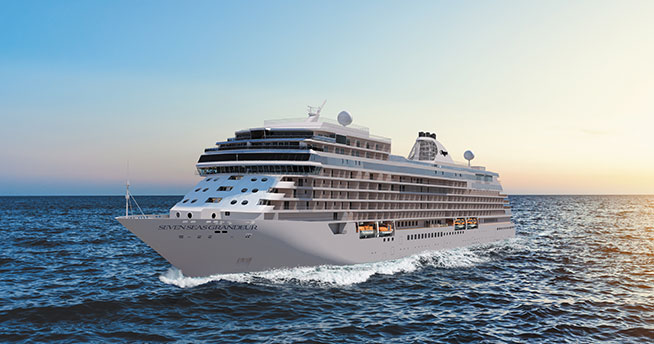This photograph, taken in landscape orientation, captures the majestic cruise ship named Seven Seas Grandeur as it sails across the blue ocean. The ship, which is primarily white with some gray hues, appears to be moving from mid-right to bottom left, cutting through slightly choppy waters. This creates a striking contrast of white waves around the vessel. The ship boasts multiple floors and balcony decks, and the image shows a mostly side view with a hint of the front. Above, the evening sky transitions smoothly from a reddish hue near the horizon to a richer blue as it ascends. The right side of the sky is brighter, indicating the sun is low and setting off-screen. The overall scene is serene yet dynamic, emphasizing both the movement of the cruise liner and the calming colors of the sea and sky.